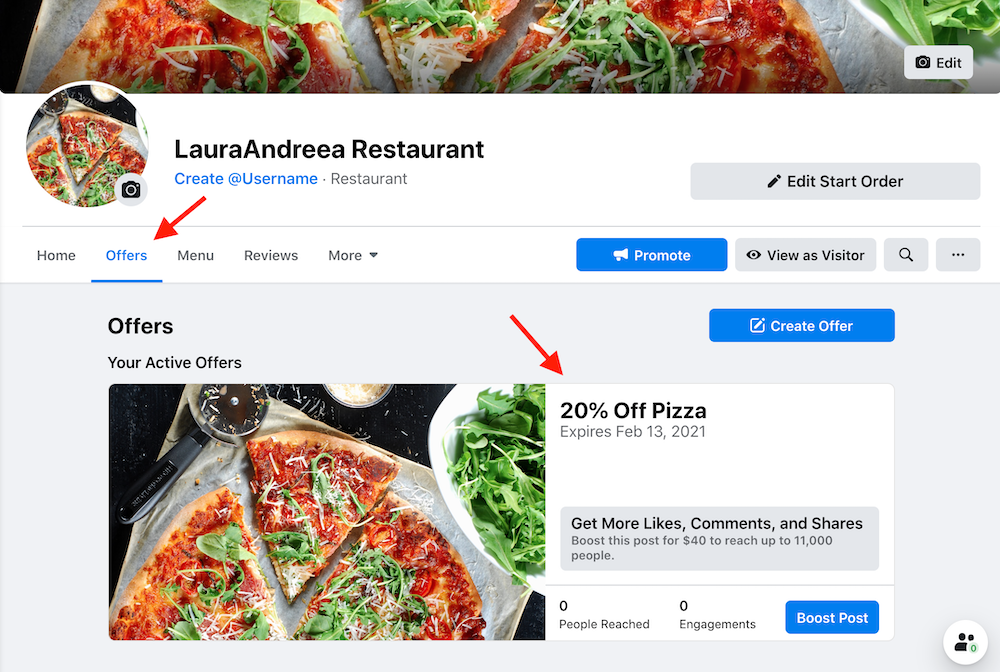A detailed screenshot showcases the Facebook business account of "Laura Andrea Restaurant." The screenshot appears to be taken from either a computer or an iPad. The account page is clearly identifiable by the classic Facebook layout and color scheme. The restaurant profile picture features an appetizing pizza. The navigation bar includes options such as Home, Offers, Menu, Reviews, and More.

A notable feature in the screenshot is the presence of red arrows pointing towards the Offers button and a specific offer: "20% off pizza, expires February 13th, 2021," indicating that the offer is outdated. Additionally, a Facebook prompt suggests boosting a post for $40 to reach up to 11,000 people, encouraging more likes, comments, and shares. The screenshot reveals options to promote the account and view it as a visitor, which means the person taking the screenshot likely has administrative access. The account hasn't created a specific username yet, and overall, the page promotes itself as a restaurant to visitors.